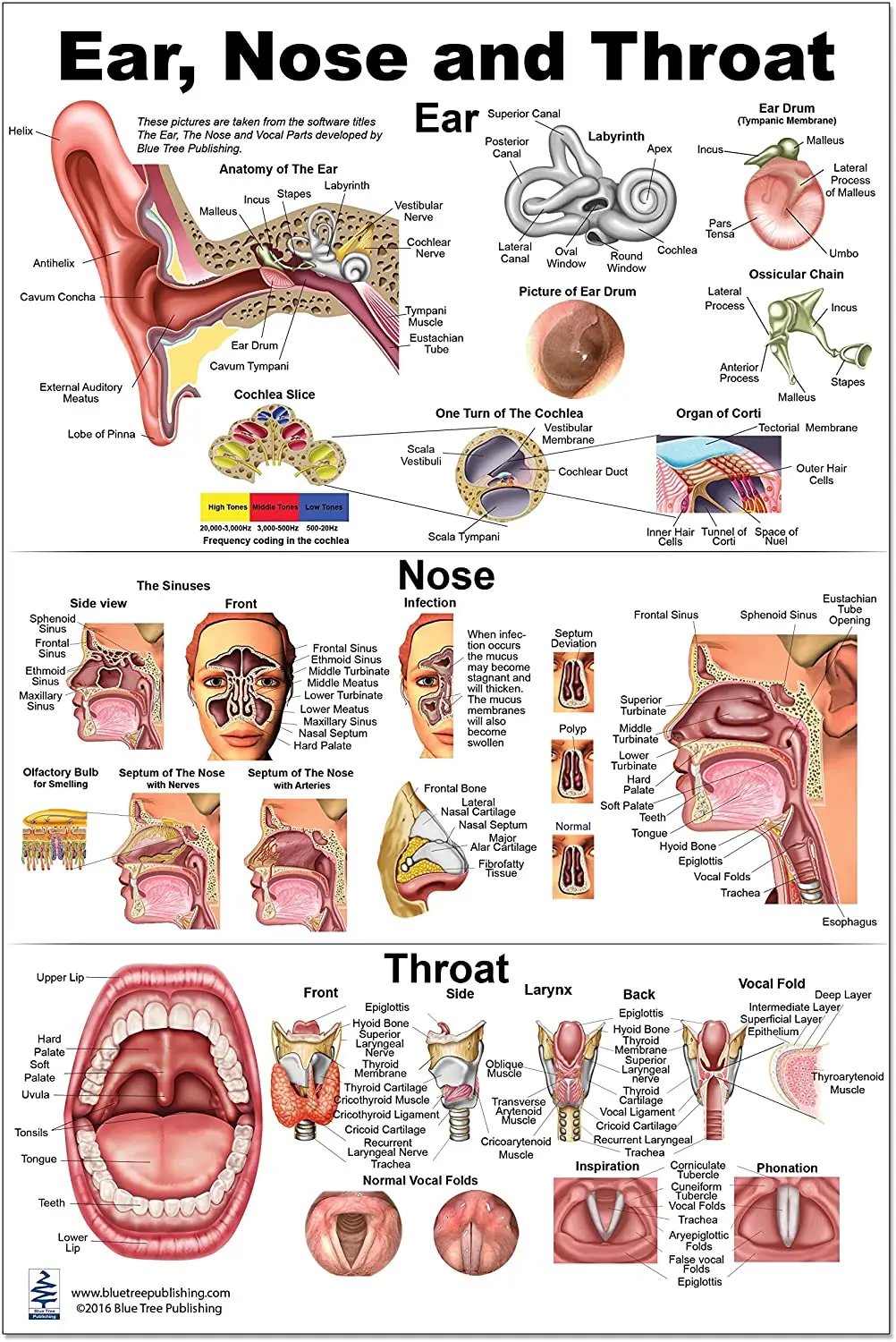This detailed medical illustration, reminiscent of educational posters found in a doctor's office, meticulously depicts the anatomy of the ear, nose, and throat against a white background. At the top, the labeled section "Ear" features a comprehensive diagram showcasing the inner workings of the ear, including an intricate portrayal of the eardrum. The middle section, labeled "Nose," includes illustrations of internal nasal structures, such as the sinuses, and features both side and frontal views of a face to highlight the nasal cavity. The bottom section, labeled "Throat," presents an open-mouth view, displaying the lips, teeth, and throat, complete with detailed labels identifying various components such as the larynx and vocal folds. The images are rendered in lifelike flesh tones, with each part meticulously annotated, making it an essential visual aid for understanding the complex anatomy of these interconnected regions.